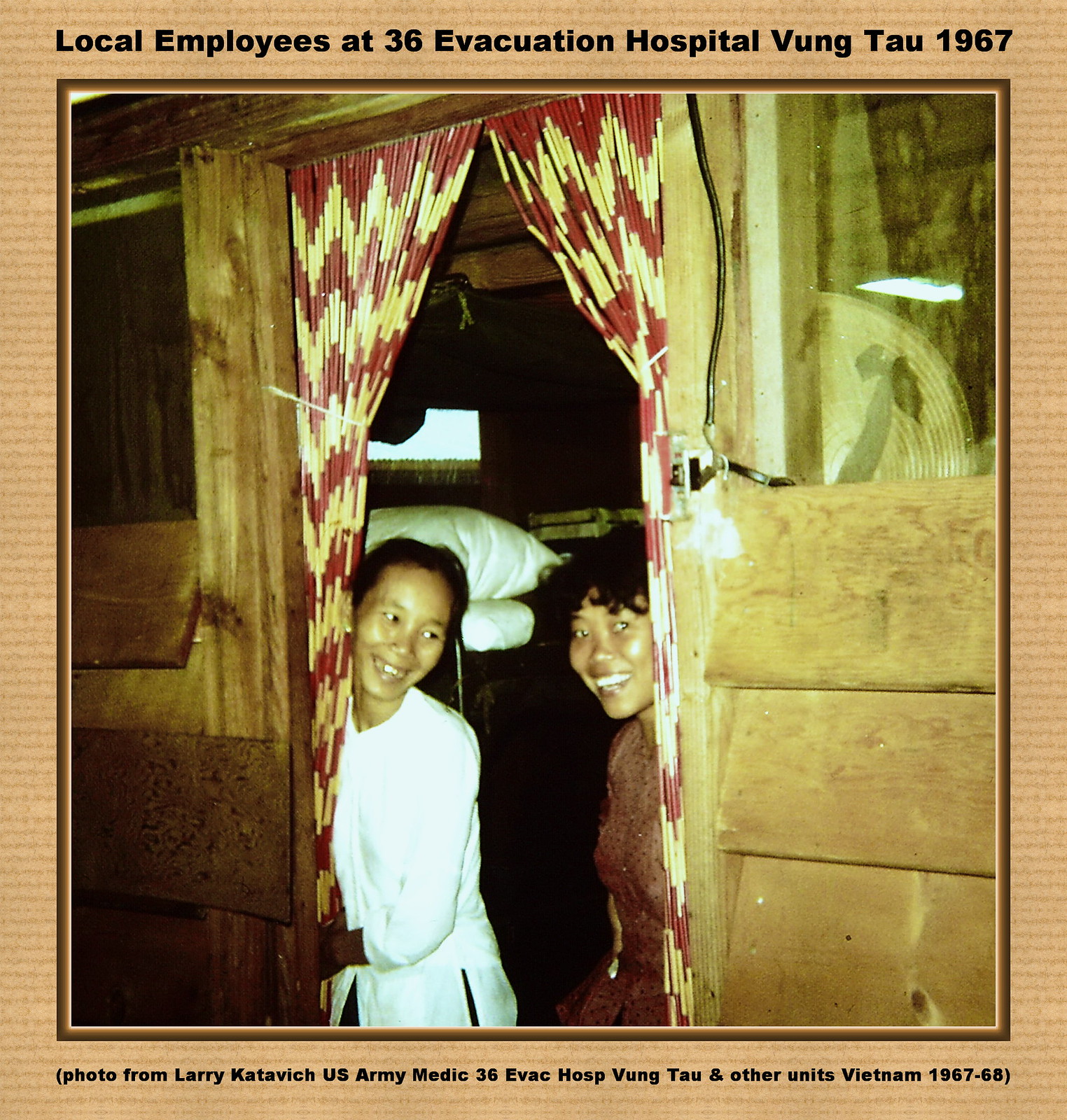The photograph captures a vibrant moment of two smiling Vietnamese women, likely local employees, inside a wooden building at the 36th Evacuation Hospital in Vung Tau, circa 1967, as indicated by the black text on the light brown background at the top of the image. Both women are standing side by side in a doorway adorned with red and yellow drapes, pulled open to reveal them. The woman on the left is dressed in white and is smiling warmly at the woman beside her, who is attired in a brown dress. Her companion reciprocates the smile, looking directly at the camera. The background reveals hints of a hospital setting, with visible pillows that suggest the presence of a cot or a bunk bed. The bottom of the image credits the photo to Larry Katovich, a U.S. Army medic at the 36th Evacuation Hospital and other units in Vietnam during 1967-68.